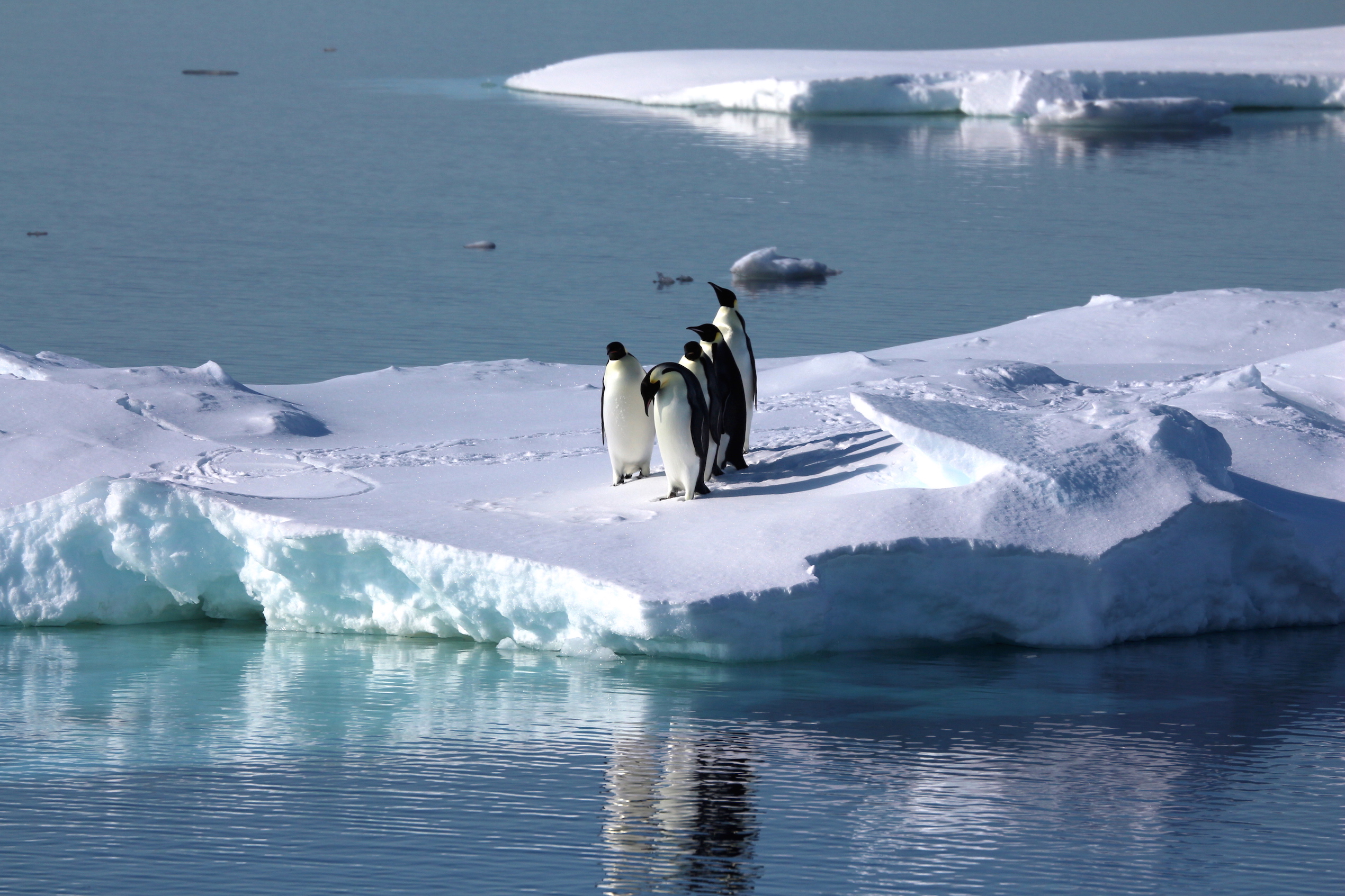The photograph captures a striking arctic or Antarctic scene on a bright, sunny day. At the center of the image, five penguins stand on a chunk of ice that juts out into the blue-green ocean. Four of the penguins are lined up in a row, facing various directions, while the fifth penguin stands slightly to the left, with its head pointed down as if inspecting the icy ground. The strong sunlight casts distinct shadows to the right of the penguins and allows their reflections to shimmer in the rippling water below. In the background, a larger ice projection looms, with a smaller iceberg floating nearby. Adding to the liveliness of the scene, a few seabirds can be seen floating on the ocean's surface, completing this picturesque and serene moment in the polar wilderness.